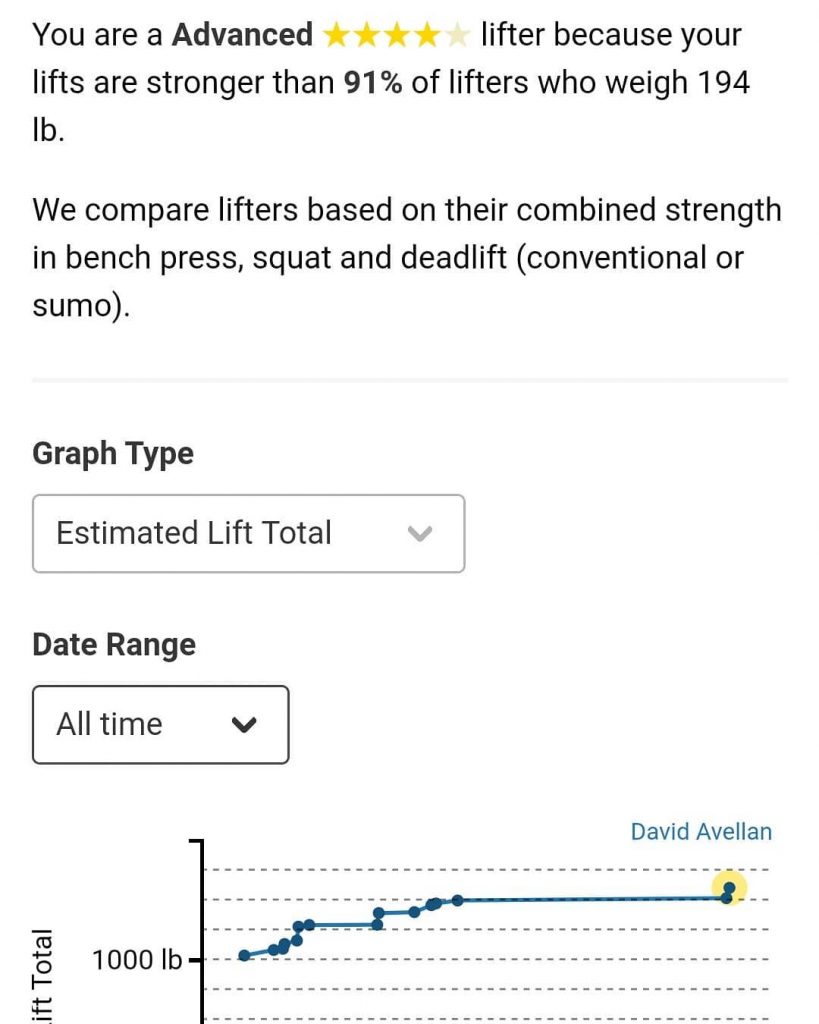The image is a screenshot from a health and fitness app. At the top, black text reads: "You are an advanced lifter because your lifts are stronger than 91% of lifters who weigh 194 pounds." The app compares lifters based on their combined strength in bench press, squat, and deadlift, including both conventional and sumo styles. Adjacent to the word "advanced," there are four illuminated yellow stars, with a fifth star not lit.

At the bottom of the screenshot, there is a blue line graph. The graph appears to compare the progress of a user named David Elavin. The left side of the graph is labeled in pounds, with the scale reaching up to 1,000 pounds. The graph's top section includes options for different graph types and date ranges. The background of the image is entirely white, providing a clean and clear context for the displayed information.